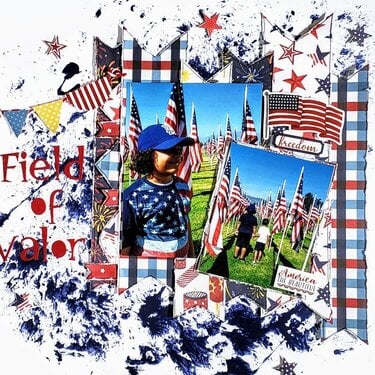The image is a scrapbook page with a patriotic theme, dominated by red, white, and blue colors. The background is primarily white, adorned with red and American flag-colored stars. Along the right-hand side, there is a vertical column of plaid in shades of red, white, and blue. In the center of the page are two photographs. The larger one features a young girl with short brown hair, smiling and wearing a blue baseball cap and a red, white, and blue American t-shirt, standing in a field filled with U.S. flags. Adjacent to this, at an angle, is a smaller photograph, showing two people with their backs to the camera, also in a field of American flags. Text on the left side of these pictures reads "Field of Valor" in red. Below the main photo, the scrapbook page has a pattern resembling blue and white waves. Other design elements include an illustration of the U.S. flag with the word "freedom" beneath it in black script on the right side, a yellow flag on the left, and various stars and banners that match the color scheme. Additionally, a white rectangle in the bottom right corner contains the words "America the Beautiful" in red and blue type. The entire layout combines color photography with graphic elements to create a cohesive, patriotic visual.